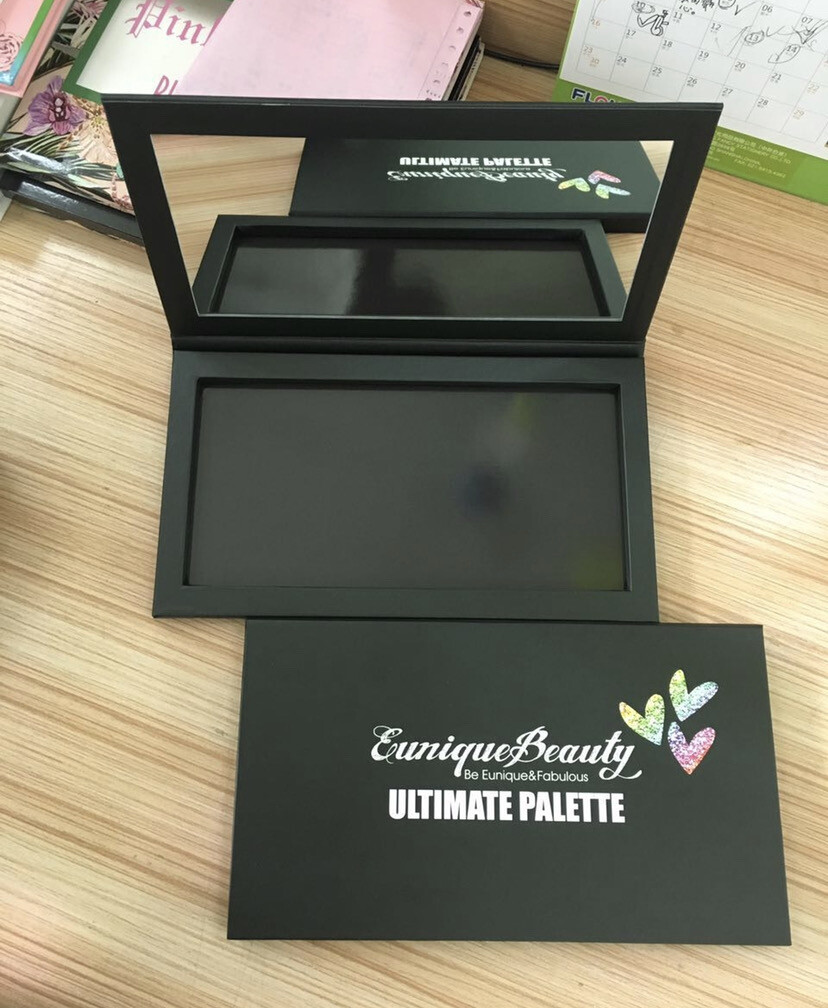In this detailed image, we see a collection of cosmetic or beauty products arranged on a wooden table, distinguishable by its straight grain. In the center of the image lies a black square object, which appears to be an open makeup palette, showcasing a mirror inside the lid. Flanking this centerpiece are two identical objects that resemble black box lids, each adorned with glitter-colored hearts in shades of yellow, green, pink, and purple. The text on these objects reads "UNIQUE BEAUTY" written in white cursive, "BY UNIQUE AND FABULOUS," and "ULTIMATE PALETTE" in bold white letters. Situated in the background, the top left corner features floral pink and green books, while the top right corner displays a calendar with a green-bordered bottom, some dates marked with indiscernible writing. The overall setting appears to be indoors, possibly suggesting a makeup room or an organized desk space.